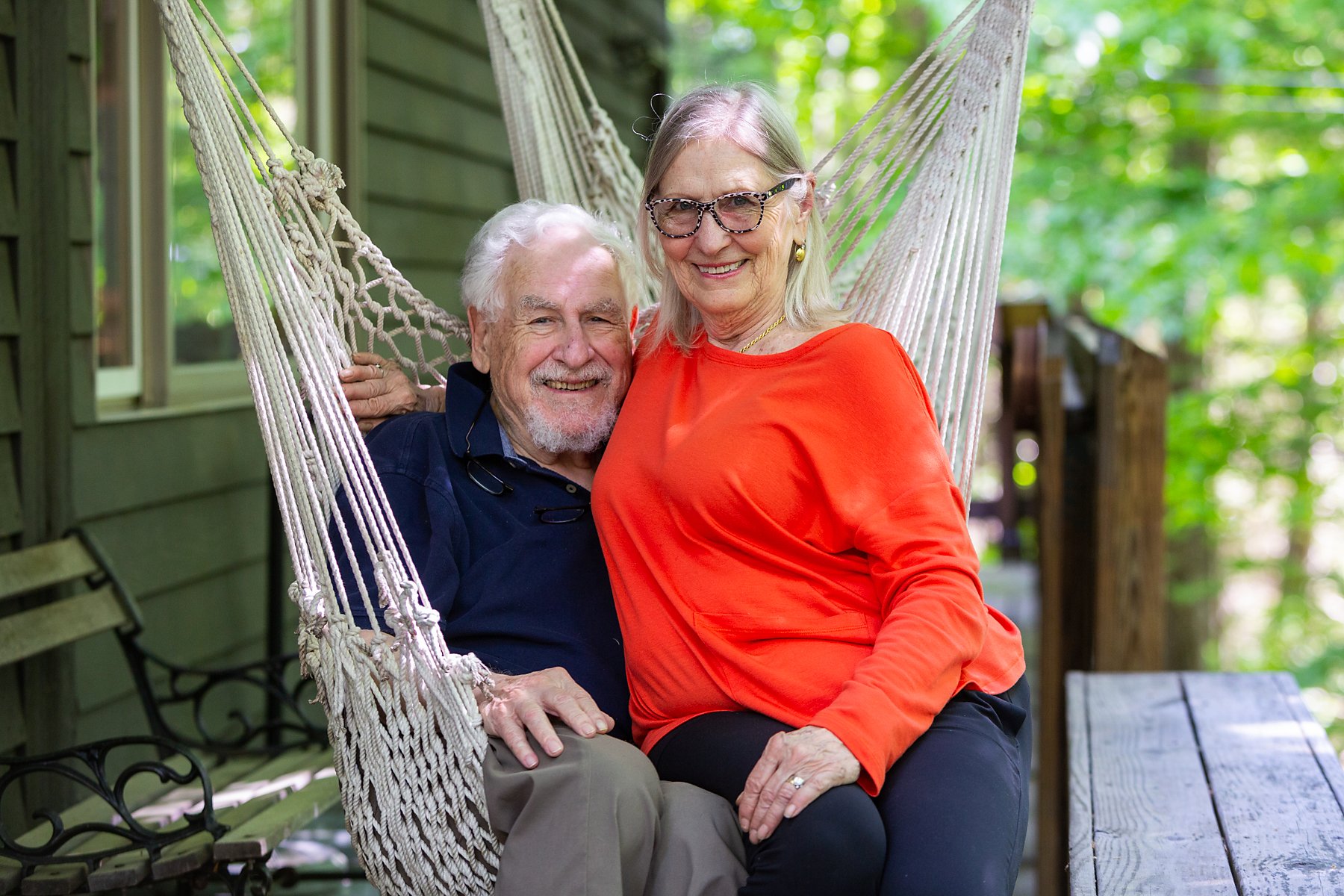In this heartwarming photograph, an older couple, appearing to be in their 60s or 70s, is captured enjoying a sunny day on the front deck of their dark hunter green house, which is surrounded by tall trees with light green leaves. They are seated in a cream-colored hammock that hangs from the ceiling of the deck. The deck also features a wooden rocking chair resting against the house walls with two white-framed windows.

The man, positioned on the left, has short white hair, a white mustache, and a beard. He's dressed in a dark blue polo shirt and gray pants, smiling warmly with his top row of teeth visible. His left hand rests on his knees. On his lap sits the woman, who has shoulder-length gray hair and is wearing brownish glasses. She is dressed in a long-sleeved orange blouse and blue jeans, also smiling widely at the camera. Both look content and joyful, suggesting a moment of shared happiness captured perfectly by the photographer.